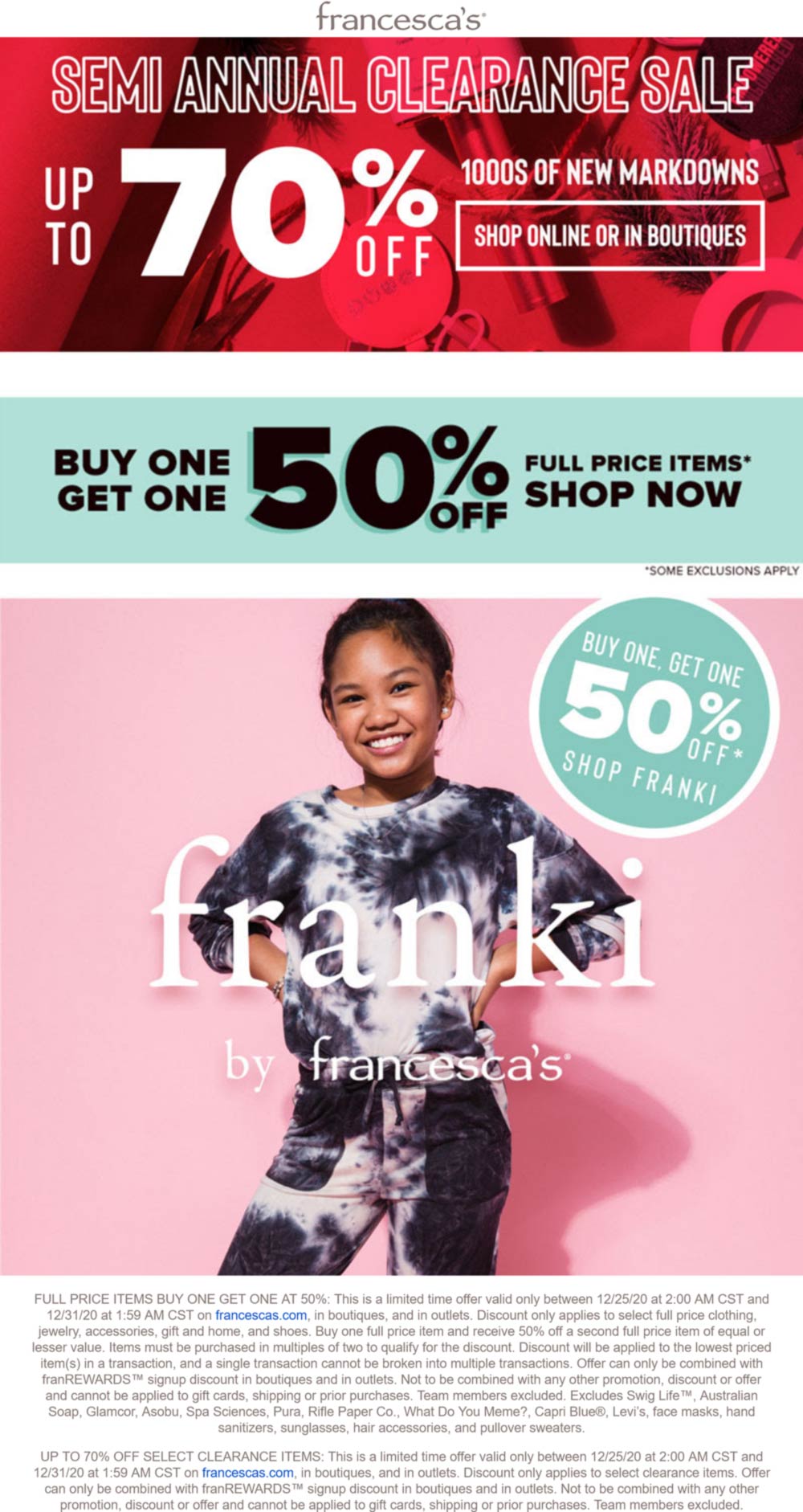The advertisement for Francesca's features a sleek and captivating design. 

At the top, "Francesca's" is displayed with a lowercase 'f' in gray, lending a modern yet minimalist appeal. Following this, a striking red and black box announces the "Semi-Annual Clearance Sale" in bold, white outlined lettering. Just below, the enticing offer "Up to 70% off" is prominently featured, accompanied by "Thousands of new markdowns" to further attract potential customers. 

The next section showcases a clean white box with the message "Shop online or in boutiques," reassuring a variety of shopping options. Beneath this, a vibrant teal box highlights another exciting deal: "Buy One, Get One 50% Off" on full-price items, urging shoppers to "Shop Now"—all in black bold lettering for maximum impact. 

Adding a touch of lifestyle imagery, the advertisement includes a picture of a girl from thigh-up, hands on her hips, donning a chic tie-dye purple and white outfit. Over her chest, the brand name "Franki" by Francesca's is stylishly presented. 

In the upper right corner, a green circle with a white border and lettering repeats the enticing "Buy One, Get One 50% Off" offer, specifically for Franki products, prompting shoppers with "Shop Franki."

Fine print at the bottom of the advertisement outlines the detailed terms and conditions of the offers. It includes specific valid dates, applicable items, and exclusions, rounding off with a mention of the additional promotion: "Up to 70% off select clearance items."

Both offers are meticulously clarified, noting that they are limited-time, valid only on francescas.com and in boutiques and outlets, and are not combinable with other promotions or discounts. This detailed and visually appealing advertisement is designed to attract and inform savvy shoppers looking for great deals at Francesca's.